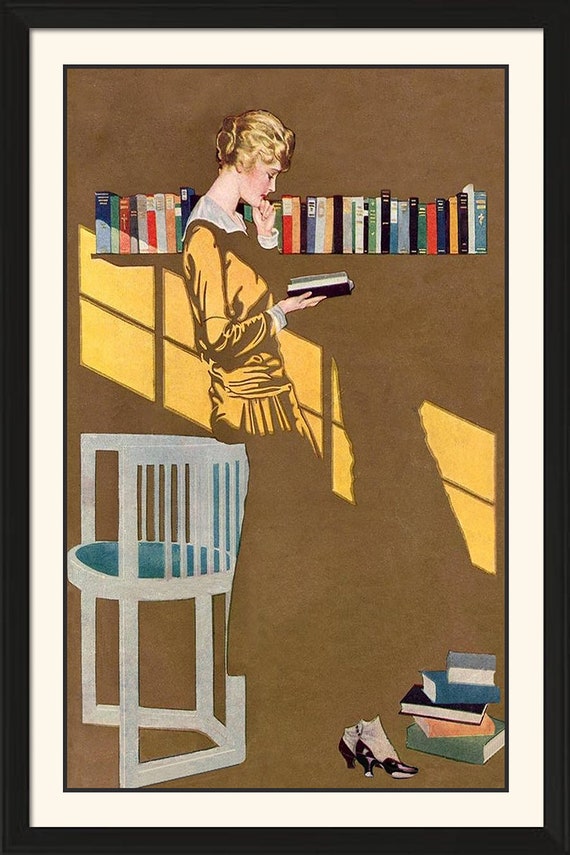The painting depicts a woman situated in a library or study, surrounded by a shelf of books. Intriguingly, the dress she wears is painted in the same color as the background wall, blending seamlessly with it. The woman is only visible where light filters through a window, casting shadows and highlighting the contours of her figure. The window frame and the play of light create a striking effect, making her dress and torso discernible in the illuminated area while the rest merges into the wall. Her feet emerge from the dress but the lower part of the garment remains indistinguishable from the background. This artwork masterfully plays with light and shadow, challenging our perception of reality and making for a fascinating visual experience.